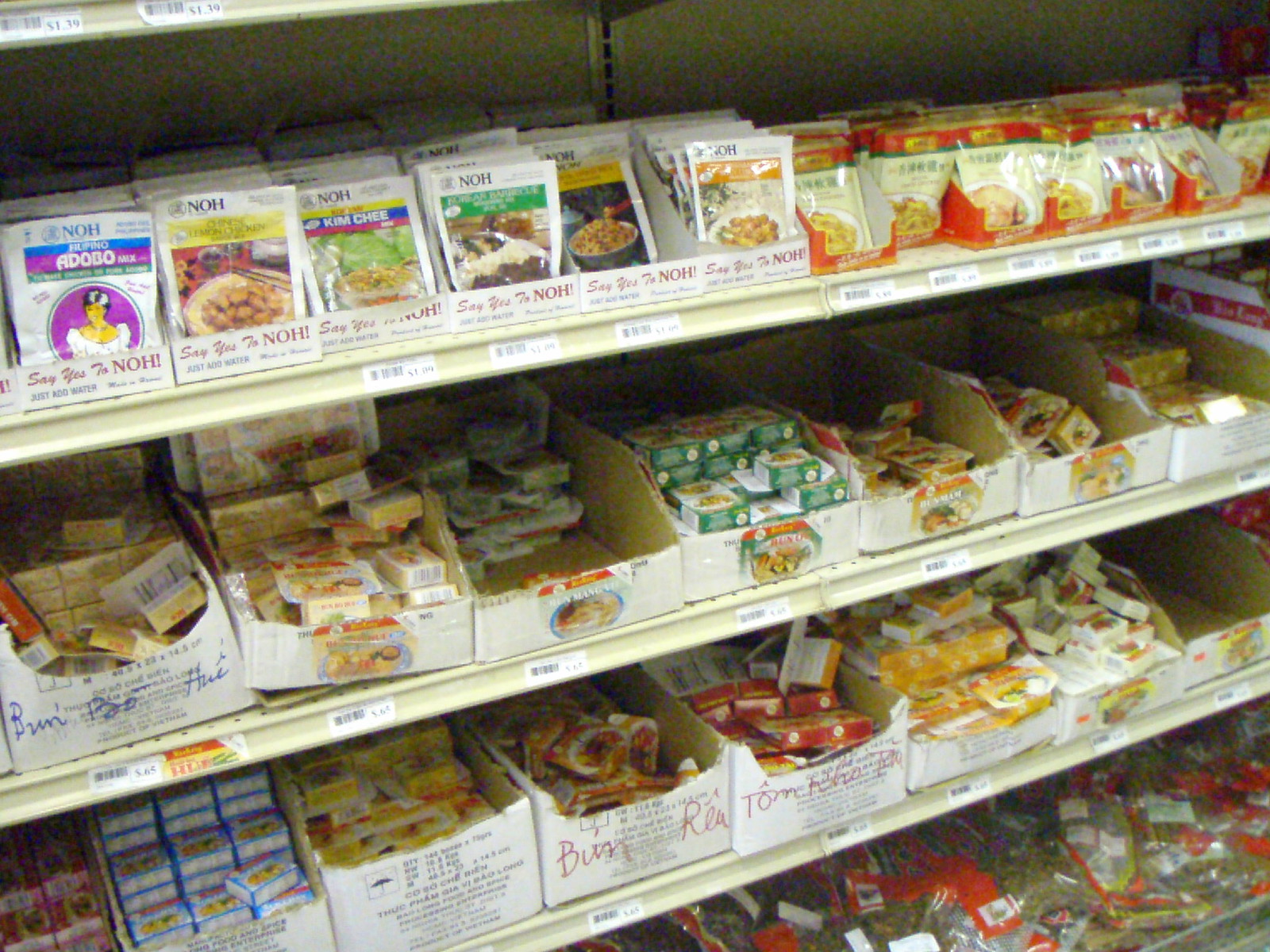The image depicts a detailed view of store shelves filled with various packaged goods. The top shelf showcases multiple envelopes, presumably containing some sort of food product, though the specific type remains unidentified. The envelopes are notable for their red stripe, followed by a thin green stripe at the top of the packaging. Moving to the second shelf, a collection of small boxes is organized, predominantly featuring yellow and white boxes alongside similarities in design with green and white boxes. A total of seven large boxes house these smaller boxes, suggesting a well-stocked inventory. The third row is a vibrant display of multicolored boxes in pink, blue, white, yellow, red, and a repeated pattern of yellow and white, adding to the variety. The lowest shelf contains several bagged or cellophane-wrapped items, marked with red and a hint of yellow, though the exact contents are indistinguishable. Overall, the shelves are meticulously stocked, offering an array of colorful and diverse goods.